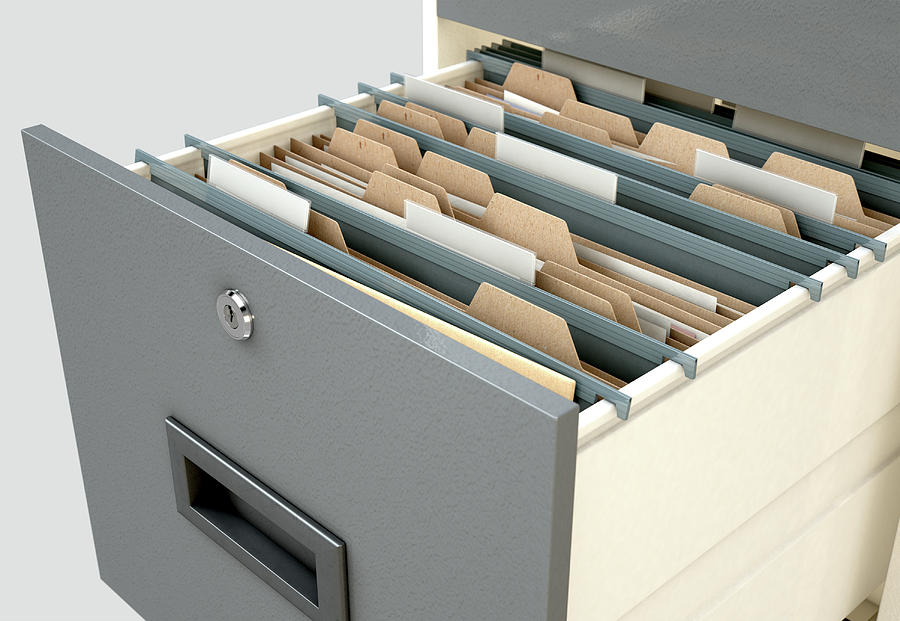In the image, we see an open drawer of a metal filing cabinet set against a light gray wall. The cabinet drawer is grayish-silver in color, likely made of metal, and features a rectangular handle for gripping and a keyhole at the top for locking or unlocking. The drawer is pulled out to reveal its contents, which include a series of hanging files. These hanging files have metal supports and appear silver on the outside, while the folders themselves are predominantly brown. Each folder has a white label at the top, but none are labeled. The view of the drawer is angled diagonally, showing the open end at the bottom left and the rest of the cabinet extending to the top right. Inside the folders, we can see slips of paper suggesting some contents, although they are not detailed or labeled.